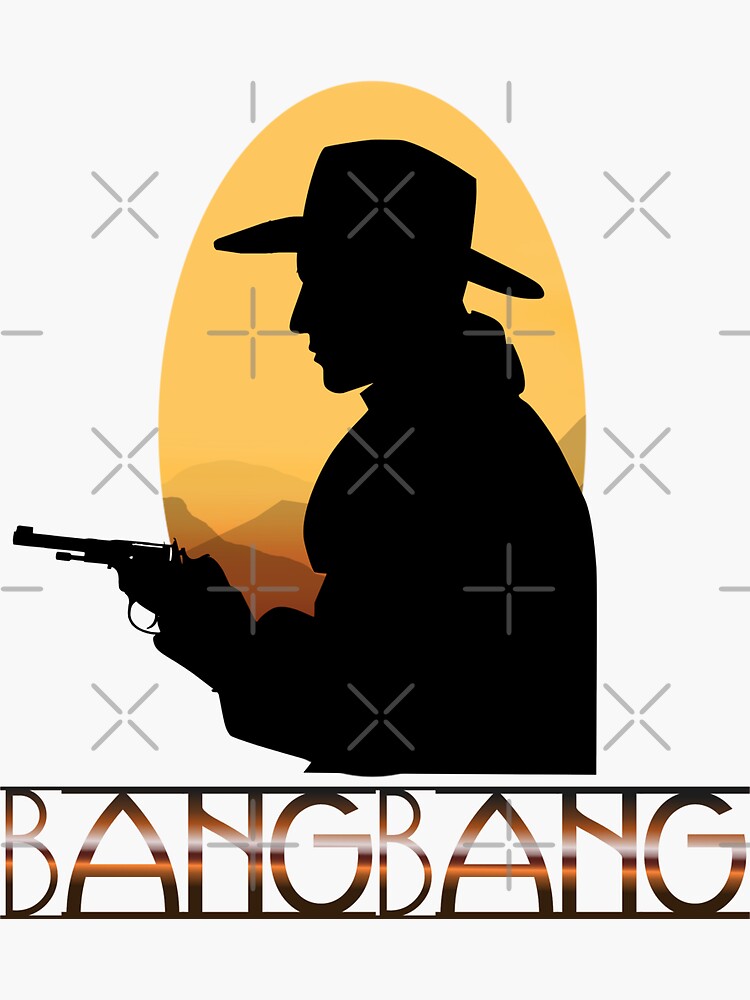The image is a vertically rectangular print with a light gray background that features faint gray X's and plus signs throughout, acting as a watermark to prevent copying. At the center of the image is an orangish oval containing a silhouette of a cowboy in profile, facing left. The cowboy, wearing a hat, has his gun drawn with the hammer pulled back, though his finger is not on the trigger. The background within the oval includes a silhouette of a mountain range in soft gradations from orange to yellow, resembling a sunset. Below the cowboy in brown lettering, enclosed by vertical lines above and below, are the words "BANG! BANG!", suggesting the sound of gunfire. Overall, the image evokes the theme of an old Western movie scene.